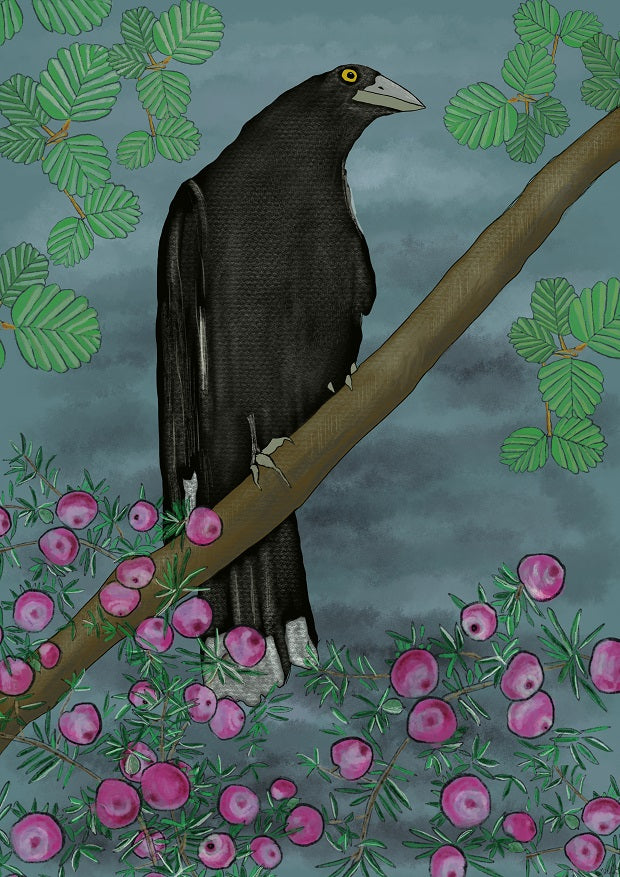The artwork is a meticulously detailed painting of a black bird perched prominently on a diagonal brown tree branch that spans from the bottom left to the top right of the portrait-oriented image. The bird, which is mostly black, features distinctive white highlights on the tips of its tail feathers and the edge of its wings. Its striking bright yellow eye is encircled by a black ring, and it has a thick, gray-white, pointy beak. The bird's talons, which appear gray or white, grip the branch tightly, giving the impression of realism with a cloth-like texture to its feathers.

The background is a nuanced blend of black and teal colors, creating a moody backdrop that contrasts with the subject. Surrounding the bird are several leaves, specifically positioned in the top left and right corners, resembling mint leaves in their small and delicate appearance. Additionally, green leaves extend from the tree branch, enhancing the natural setting. Toward the bottom of the painting, clusters of round, pinkish-purple berries with thin leaves add a vibrant detail, hanging from brown vines intertwined around the lower branches. Gray clouds linger in the background, further enriching the scene with an atmospheric depth.